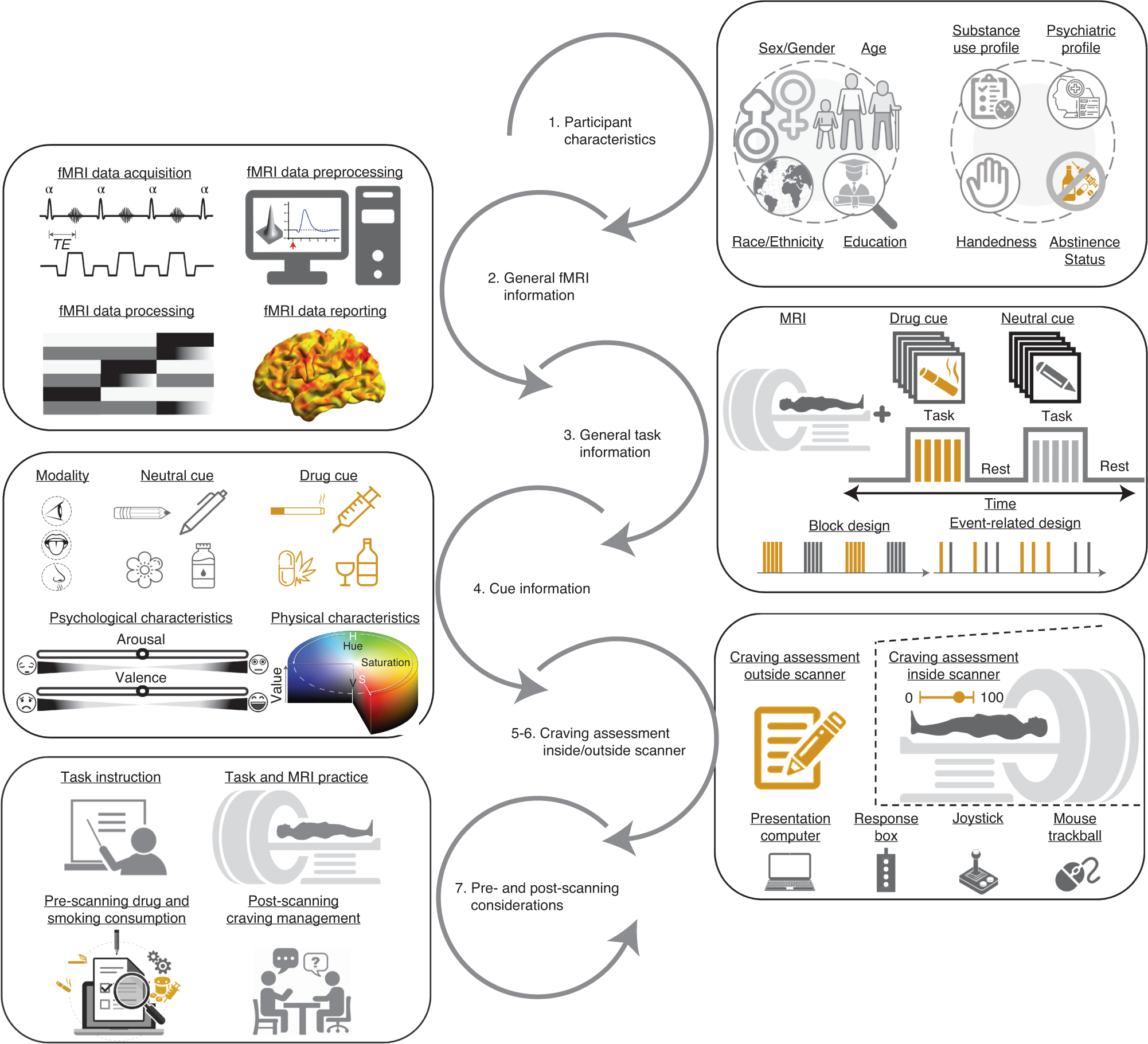The image is a detailed flow chart illustrating the comprehensive process involved in fMRI studies. The chart includes various black lines of text accompanied by relevant images. Starting from the left, the text sequentially reads: "fMRI data acquisition," "fMRI data preprocessing," "fMRI data processing," and "fMRI data reporting."

On both sides of multiple curved lines, there are three rectangles. These rectangles cover diverse aspects, such as modality, cue types (neutral and drug cues), and participant characteristics. The chart is segmented into seven distinct parts, each with arrows pointing downward to indicate the flow:

1. **Participant Characteristics** - Detailing demographic aspects such as sex, gender, age, race, ethnicity, education, substance use profile, psychiatric profile, handedness, and abstinence status.
2. **General fMRI Information**.
3. **General Task Information**.
4. **Cue Information** - Differentiating between neutral and drug cues.
5-6. **Craving Assessment Inside/Outside Scanner**.
7. **Pre- and Post-Scanning Considerations**.

The right side of the image includes visual depictions like bar charts on a computer monitor, a multi-colored brain image with yellows, oranges, and reds, and symbols representing various stages of the fMRI process, including modality, arousal, valence, physical characteristics (hue, saturation), task instructions, pre-scanning drug and smoking consumption, and post-scanning craving management.

Silhouettes of people and icons representing different tasks and MRI procedures further elaborate on the detailed steps from data acquisition to data reporting, emphasizing the meticulous and comprehensive nature of fMRI study protocols.